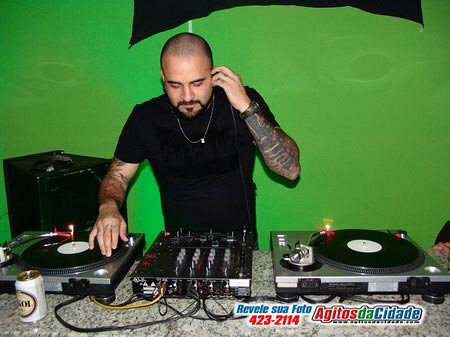The image depicts a DJ setup with a man standing in front of a large green background wall. Centrally positioned are two record players, one on his left and one on his right, both with records on them. Between the turntables lies a six-function mixing board, full of switches and numerous wires visible in front of the equipment. The DJ, wearing a black T-shirt and a gold chain, is actively scratching a record with his right hand while holding an earphone to his ear with his heavily tattooed left arm. His right arm also shows some tattoos. The DJ has a shaved head, a goatee, and a thin mustache. In the front left corner, a can of beer is noticeable. Below the setup, there's an advertisement featuring the text "Reverly Suatorto" along with a phone number and the name "Aquitas de Cidade."